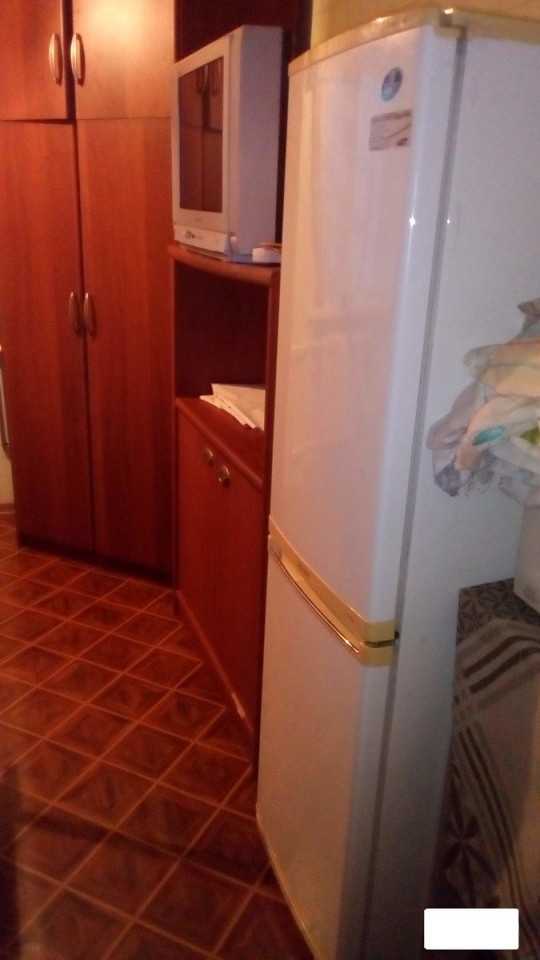This photograph depicts a combined kitchen and living space with a distinct layout and dated decor. The flooring is a less expensive brown linoleum with a square design, resembling wood tiles, giving a somewhat rugged appearance. A prominent feature is the tall, white refrigerator with a freezer section on the bottom. The fridge is adorned with a brown-blue sticker and a square-red sticker on the top right.

Adjacent to the refrigerator is a wooden built-in cabinet that houses an older model flat-screen TV, hinting at a design from around 10 years ago, still somewhat thick by modern standards. Below the TV, the cabinet features an open shelf cluttered with stacks of paper, and at the very bottom, it has two wooden doors offering additional storage.

The area seems multifunctional, possibly an employee room, due to the unconventional mix of appliances and media. Beside the cabinet, there is another tall structure with sets of cabinets; two more doors at the bottom and shorter, higher cabinets on top. The scene is dimly lit with a warm ambiance, adding to the cozy, albeit slightly cluttered feel of the space.